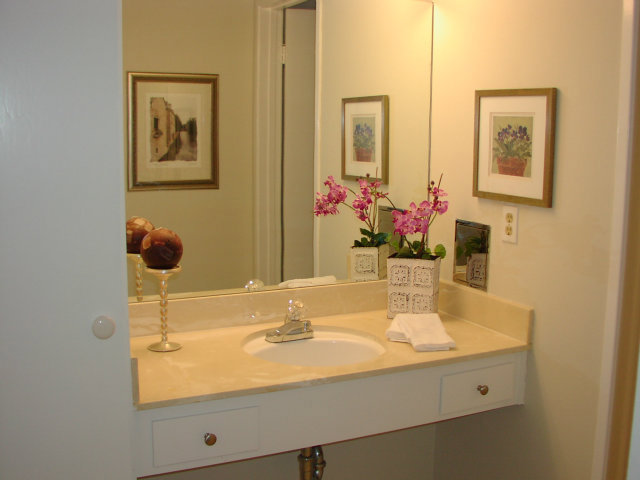This photograph showcases a meticulously neat and modern bathroom. The primary focus is on a stylish sink with a flat beige countertop and a white basin integrated into its center. The sink features a sleek silver faucet with a transparent handle for operation. To the left of the sink stands a tall, wine glass-shaped silver ornament topped with a brown sphere, adding an artistic touch. On the right side, two neatly folded white hand towels are placed beside a rectangular white pot containing vibrant pink orchids with lush green leaves. 

Above the sink, the spotlessly clean bathroom mirror is framed in an elegant golden border, reflecting the wall behind it. This wall displays a picture in a brown wooden frame, depicting a potted plant with purple flowers, adding a natural and vibrant element to the space. Below the countertop, the area is kept minimalist with visible silver piping against the pristine white walls, enhancing the room's modern aesthetic.